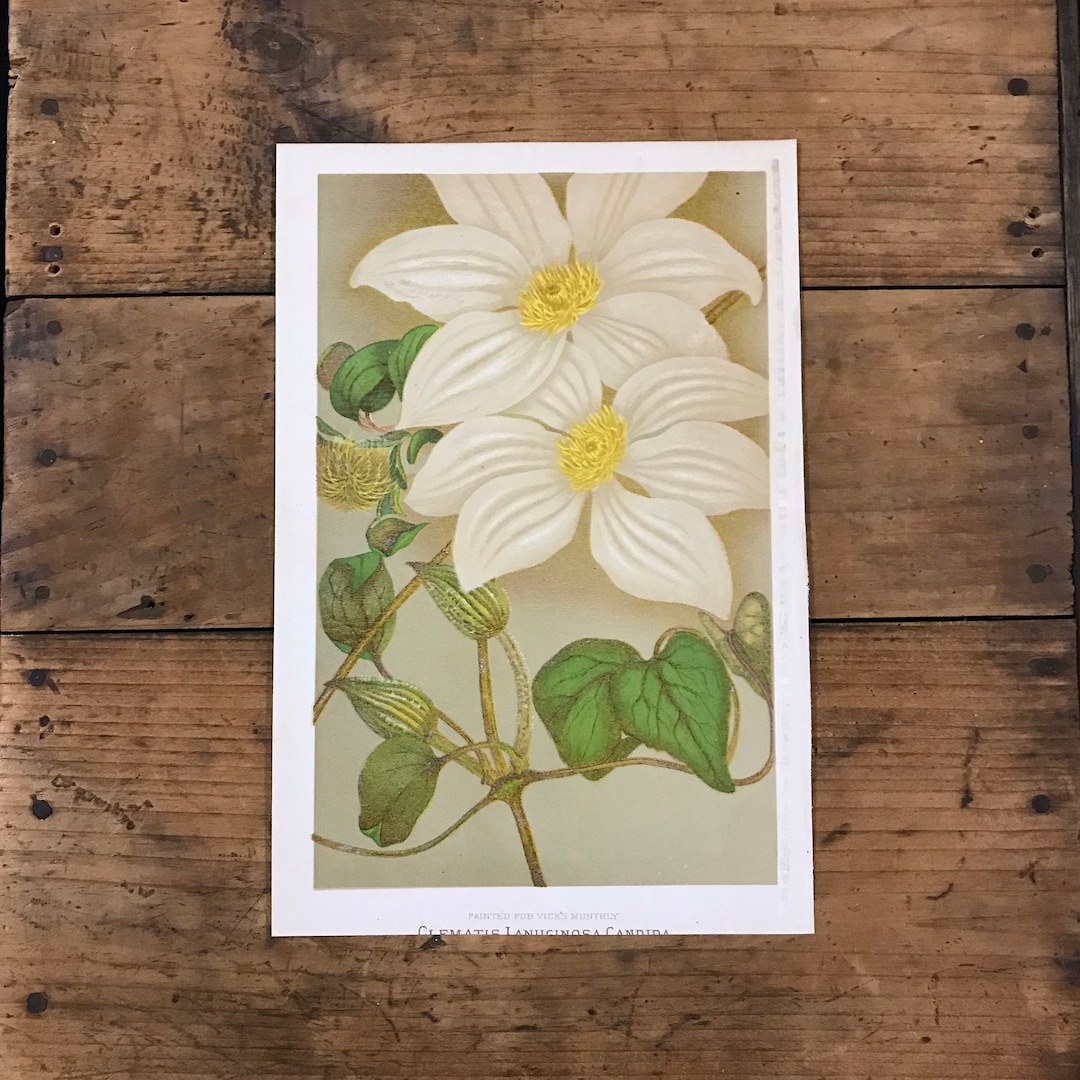The image features a card with a white frame, mounted on a rustic, weathered wooden wall adorned with visible nail holes and scratches, which gives it a barn-like appearance. The card itself showcases two white flowers, each having six petals that narrow at the base, widen in the middle, and taper to a point. Both flowers have vibrant yellow centers. Below the flowers, there are buds yet to bloom, promising to produce more flowers. Surrounding the flowers are heart-shaped green leaves with vein-like patterns in a darker shade, and a tan-colored stem speckled with black. Additionally, a green butterfly flutters near one of the leaves. The bottom of the card contains partially visible text that reads "Clematis Lanuginosa Candida."